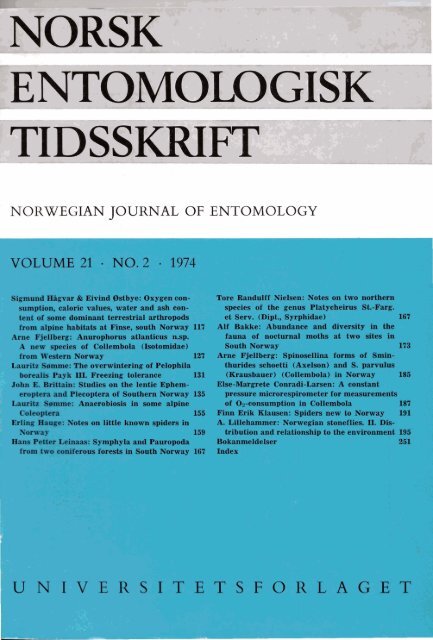The image appears to be the cover of an issue of the Norwegian Journal of Entomology, specifically Volume 21, Number 2, from 1974. At the top, three gray rectangles contain the title in Norwegian: "Norsk Entomologisk Tidskrift," written in black text. Below these rectangles, a white section features the English translation, "Norwegian Journal of Entomology," also in black text. The bottom part of the cover is a teal-blue square containing two paragraphs of small black text outlining the table of contents and listing the articles along with their corresponding page numbers. At the top of this teal section, it states in black text, "Volume 21, Number 2, 1974." At the very bottom, the text reads "Universitet for LaGette," though the exact spelling is somewhat unclear. The visual presentation and font styles suggest that this is a scholarly publication, likely linked to a university or academic institution.